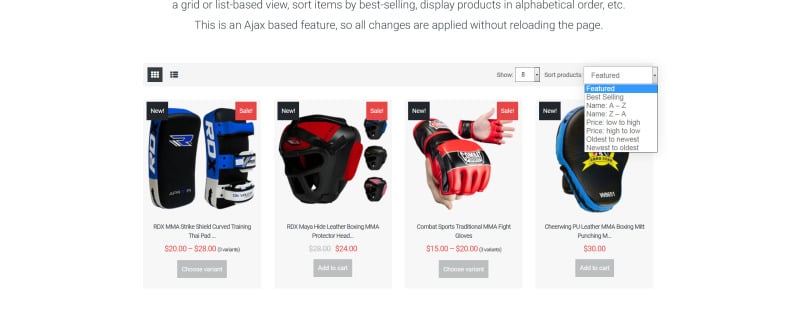The web page displays various MMA training products with features for sorting and filtering. At the top, there is black text that outlines options such as grid or list-based views, sorting by best-selling, and displaying products in alphabetical order. These features are Ajax-based, allowing changes without page reloads.

On the left, there are RDX MMA strike shields in two styles: one black on the front with blue edges, and another with blue sides. The text reads "RDX MMA Strike Shield Curved Training Thai Pad..." in black, followed by the price range in red, "$20 to $28." Below this is a dark gray button with white text that says "Choose Variant."

Next is the RDX Mayo Hide Leather Boxing MMA Protector Headgear, primarily red with black detailing. Its original price of $28 is crossed out in gray, with a new price of $24 in red. A dark gray "Add to Cart" button with white text is below this item.

To the right are red and black combat gloves that cover the top of the hand but leave the palm exposed. This product features a black "New!" button and a red "Sale!" button. Beneath the gloves is the label "Combat Sports Traditional MMA Fight Gloves," priced between $15 to $20, with "three variants" noted in black text. There is also a "Choose Variant" button.

Top-right on the page, there is a dropdown showing a list of 5 items by default, and another dropdown for sorting products, with "Featured" currently selected. Other sorting options include best-selling, name A to Z, name Z to A, price low to high, price high to low, oldest to newest, and newest to oldest.

Finally, a black boxing pad with a yellow circle marked with dark blue text is displayed. The edges are also dark blue and the text reads "Cheer Wing PU Leather MMA Boxing Mitt Punching..." in all caps. This item is priced at $30 with a dark gray "Add to Cart" button in white text below.